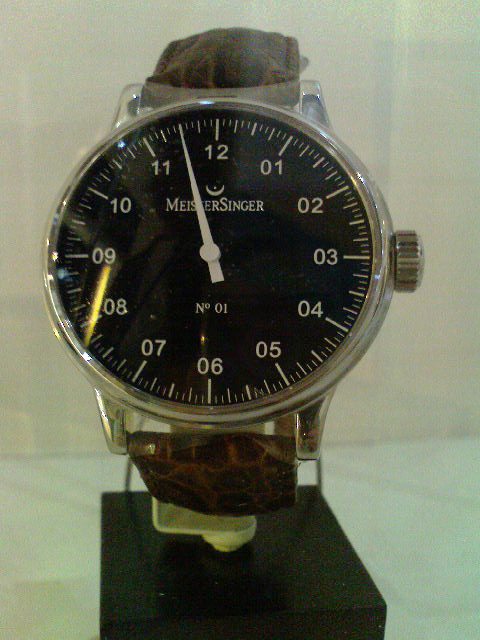This is a detailed close-up photograph of a uniquely designed watch, distinctively resting on a clear plastic stand that sits atop a small, black wooden pedestal. The background is gray, and the counter beneath is white. The watch, crafted by the brand Meistersinger, features a durable brown leather band with a textured reptilian look, possibly resembling alligator or snake skin. The watch itself has a sleek silver casing and an all-black face complemented by simple yet striking white numerals, each prefixed with a zero for a unique touch, such as "01," "02," and so on, extending from 12 to 11 with minute markings and even smaller ones in between. Notably, the watch displays only a singular white hand, pointing between the 11 and 12, suggesting the time might be around 11:50. There is a silver winding knob on its right side. The design of this Meistersinger timepiece emphasizes both minimalist and avant-garde elements, making it an intriguing and stylish accessory.